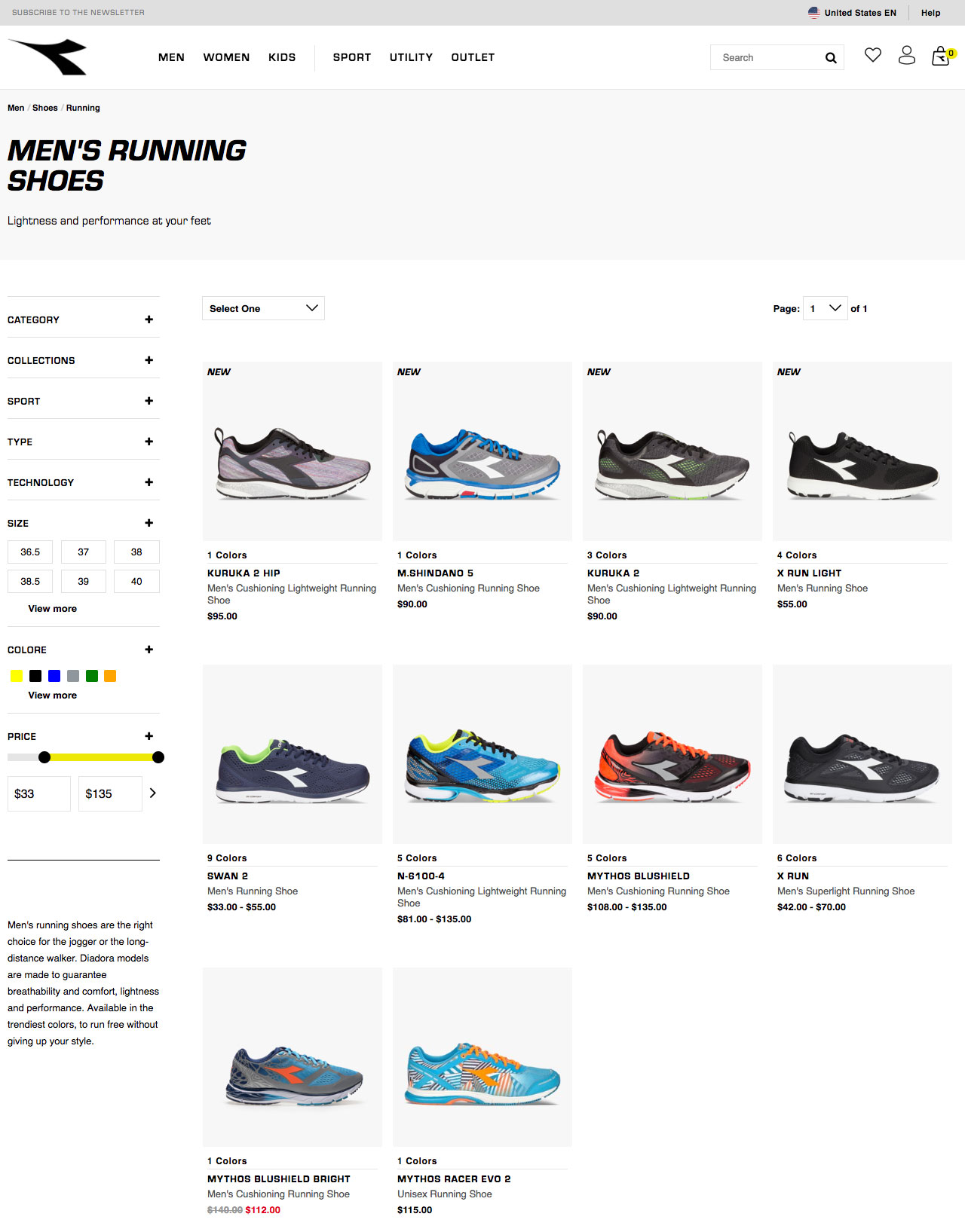The image features a detailed webpage layout designed for shopping. At the very top, a white background dominates the scene, except for a small gray box containing extremely tiny text on both the left and right sides. Below this, there's another white box displaying a black mark shaped like a sideways V. 

Continuing down, various navigation options are listed, including "Men," "Women," "Kids," "Sport," "Utility," and "Outlet". To the right of these, there is a search bar, a heart icon, a user icon, and a battery icon with a tiny yellow dot beside it.

The main section of the page has a light blue background with some text; prominently, it reads "Men’s Running Shoes," accompanied by some smaller text below it. 

Further down, the white background returns, housing several small boxes each marked with a plus sign. These seem to be category and selection filters. There’s also a size filter displaying six size options, along with a "View More" button. A color filter is present with various color options including yellow, black, blue, gray, green, and orange, each accompanied by a plus sign for further selection.

Beneath the color options, a price filter appears, featuring a slider marked with yellow and black dots, ranging from $35 to $136. 

On the right side of the page, there's a 'Select one' dropdown box with a down arrow. Below this dropdown, ten images of different shoes, each accompanied by detailed descriptions, are displayed.